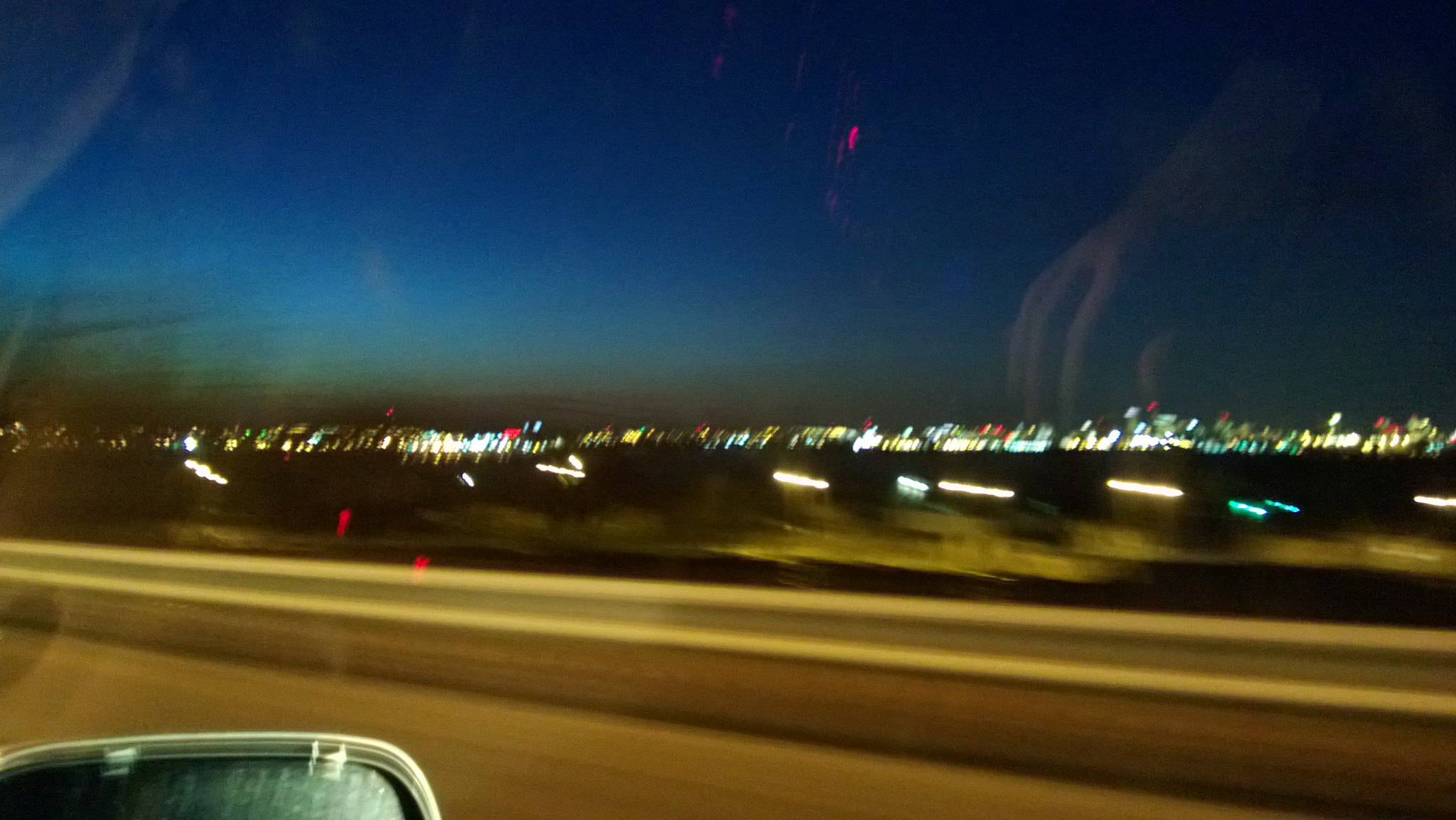The image is a nighttime photograph taken from the front passenger seat of a moving car. The picture captures the scene through the car window, featuring a blurred background indicative of motion. In the lower right corner, the top of a streaked and dirty rearview mirror is visible. Outside the window, a gray guardrail runs horizontally across the center of the image. Above the guardrail, the city lights, possibly including building and stadium lights, are blurred due to the car’s movement. The dark blue sky transitions to a lighter shade towards the horizon on the left side of the image. Reflecting in the window, the faint outline of a hand from the person inside the car can be seen superimposed over the scene.